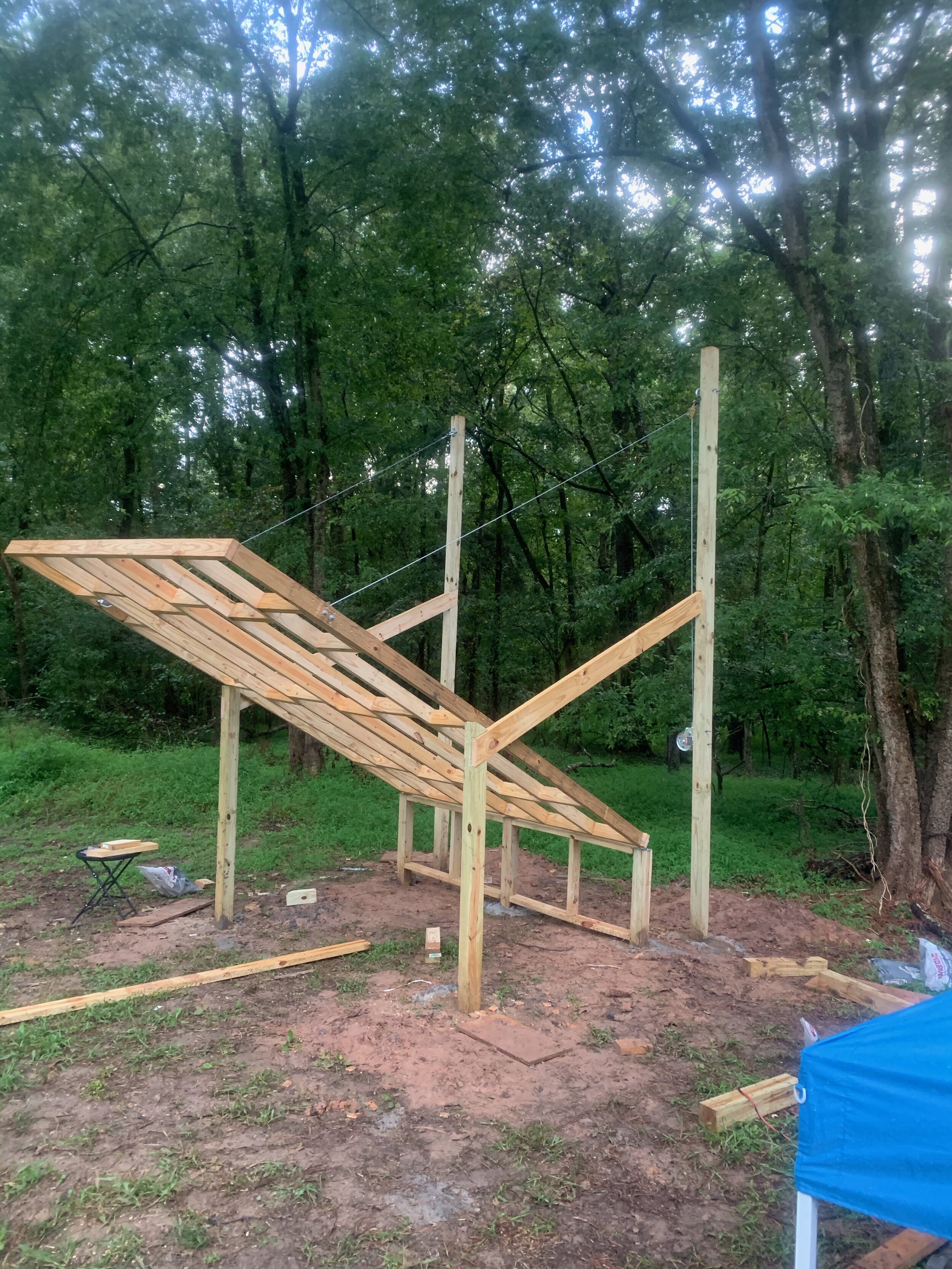In this vertically aligned rectangular picture taken outdoors, we observe a rustic wooden structure set amidst a natural backyard setting. At the top of the image, tall trees with green leaves punctuate the scene, their branches revealing patches of blue sky and luminous white clouds. Descending into the middle of the frame, a humble backyard landscape transitions from green grass to a foreground dominated by brown dirt with a few sprouting weeds. 

Central to the image, a wooden frame with numerous square cutouts is suspended at a diagonal angle by taut cords connected to vertical wooden poles at each end. This frame leans from the bottom middle towards the upper middle left of the picture and rests on the earthy ground. Notably, a separate wooden post lies horizontally on the ground nearby. 

In the lower right corner, a white leg and tightly wrapped blue fabric suggest the presence of a structure, possibly a table or a pop-up tent, adding a subtle human element to the serene outdoor scene.